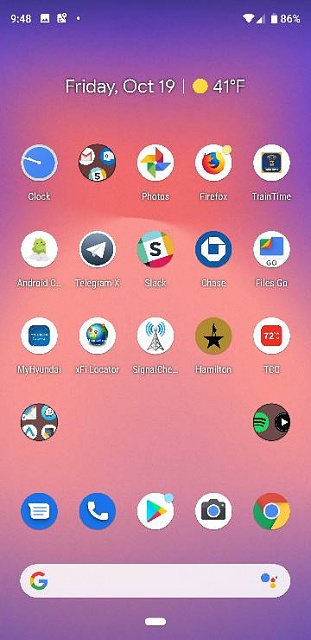This is a detailed screenshot of a mobile device's home screen. The background features a gradient with purple around the edges and a striking pink spot at the center. The app icons are meticulously organized into a 5x5 grid. At the bottom, a white Google search bar adorned with the colorful 'G' logo on the left is prominently displayed. The status bar at the top provides essential information such as the time, running background apps, and indicators for WiFi, network signal strength, and battery level. Directly beneath this bar, the date—Friday, October 19th—and the weather are shown, with the temperature being 41°F represented by a round yellow circle symbolizing the sun. The app icons are arranged as follows: the first row includes the clock app; the second row holds various messaging apps; the third row contains the photos app; the fourth row features Firefox; and the fifth row is dedicated to the Train Time app.